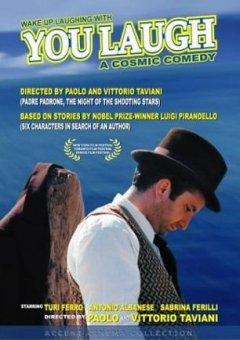This highly detailed movie poster, advertising the film "You Laugh," presents an intriguing blend of visuals and text against a blue ocean-like background. At the very top, the text reads, "Wake up laughing with You Laugh, a cosmic comedy," setting a playful and whimsical tone for the film. The poster credits Paolo and Vittorio Taviani as directors and mentions it is based on stories by Nobel Prize-winning author Luigi Pirandello, with an additional reference to "The Night of the Shooting Stars" and "Six Characters in Search of an Author." 

Prominently positioned towards the bottom right of the poster, a man with a light skin tone is shown in profile. He wears a black dressy hat, a white dress shirt, a gray patterned vest, and a black tie. His short, dark hair almost blends into the hat as he looks down pensively. Meanwhile, on the bottom left of the poster, a large rock partially submerged in the ocean adds to the atmospheric setting. The names of the starring actors, Terry Farrow, Antonio Albany, and Sabrina Farrelly, are listed at the bottom, re-emphasizing the direction by Paolo and Vittorio Taviani. The entire composition exudes a sense of dramatic yet comedic storytelling.